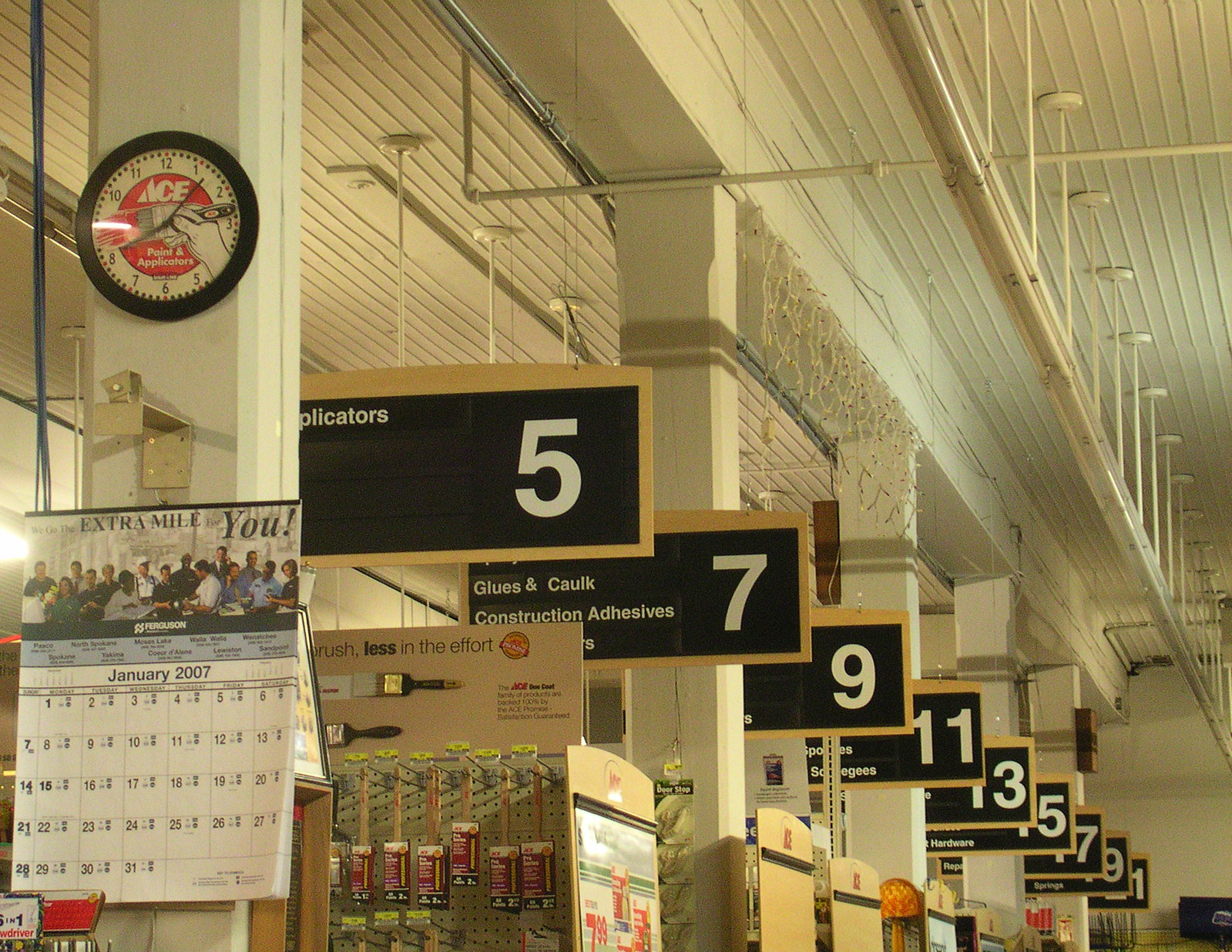The indoor color photograph captures the intricate details of an Ace Hardware store. The focal point is a series of rectangular, black aisle signs with white lettering, displaying odd-numbered aisles in ascending order: 5, 7, 9, 11, 13, 15, 17, 19, and 21. These signs hang diagonally from the left of center towards the background on the right, suspended from the ceiling. Below the signs, the ends of the aisles are visible.

On the left side of the image, a white support column is prominent. Halfway up this column hangs a calendar which features a motivational message, “Extra mile for you” and shows the month of January 2007, along with a photograph of a group of people. Above the calendar is a metal bracket, and further above, a round wall clock is positioned. The clock reads six minutes past eight and displays the Ace logo below the twelve o'clock position. Additionally, the clock face intriguingly shows a hand holding a paintbrush coming from the four o'clock position.

The ceiling of the store is white and features visible pipework and fluorescent lighting that stretches diagonally from the top right to the lower right edge, although the lights are not illuminated. Scattered holiday decorations remain, indicative of the recent Christmas season. The scene is rich in hardware store ambience, with examples such as “Applicators” in aisle 5 and “Glues and Caulk” in aisle 7, further enhancing the detailed narrative of the hardware-filled environment.